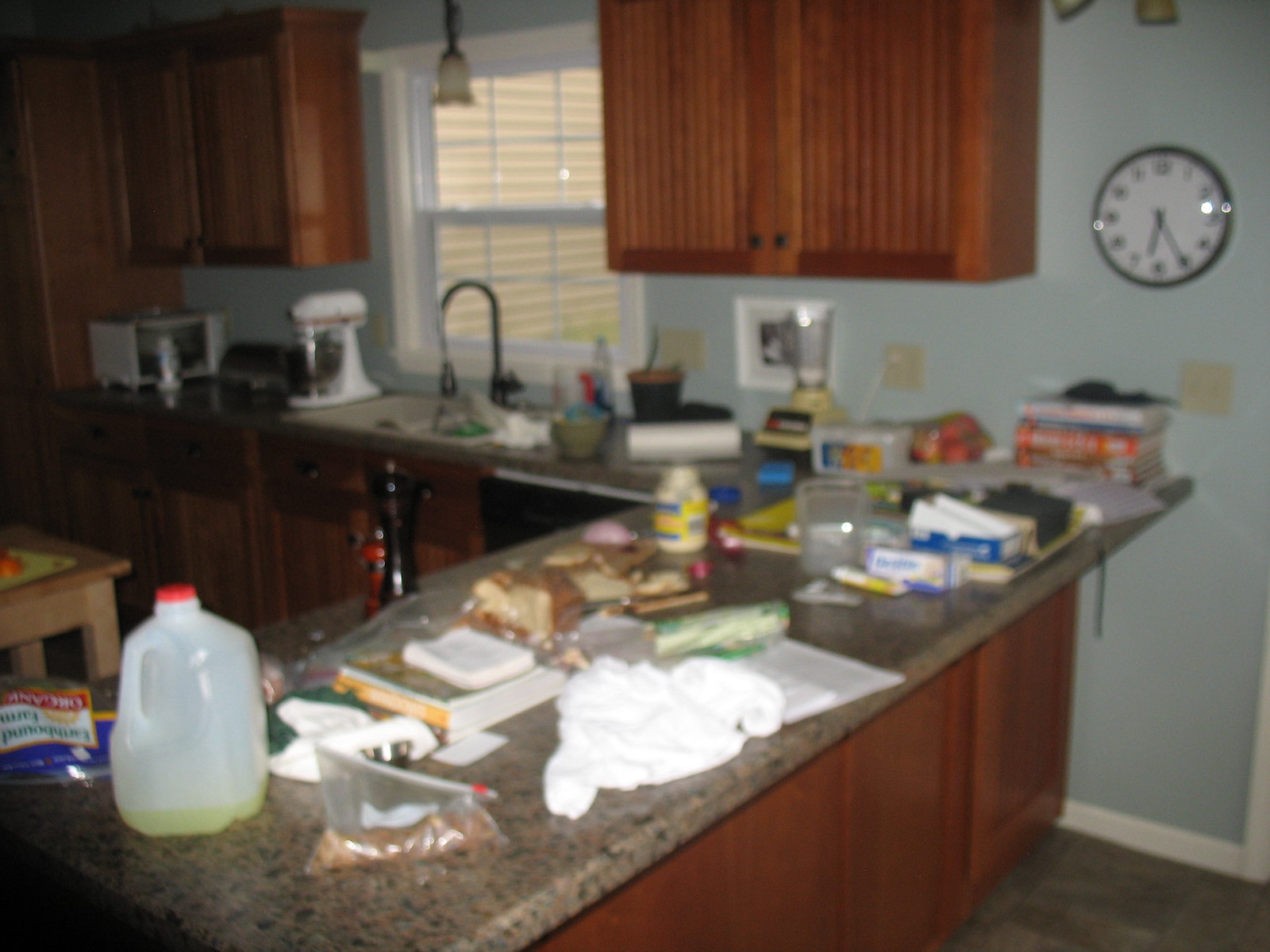A blurry image depicts the cluttered interior of a kitchen. Dominating the background is a pale blue, almost baby blue wall that features a white analog clock with a black border. Attached to this wall is a series of brown cabinets, complemented by a white window divided by a vertical white bar. More cabinets are positioned behind and extend down to meet an L-shaped countertop. This countertop, made of a gray marble-like surface, stretches from the back of the wall and juts out towards the bottom left corner of the image. Below these cabinets, additional sections of wooden paneling are visible.

In the center, there is a light wooden table. The L-shaped countertop is cluttered with various items: a jug that appears to contain cooking oil, several plastic bags, scattered slices of sandwich bread, books, a towel, a jar of mayonnaise, and various blue boxes and containers. A stack of books rests against the wall, along with a blender and a roll of toilet paper. In the far back, a kitchen mixer and a microwave can be seen, alongside a sink equipped with a large curved black faucet.